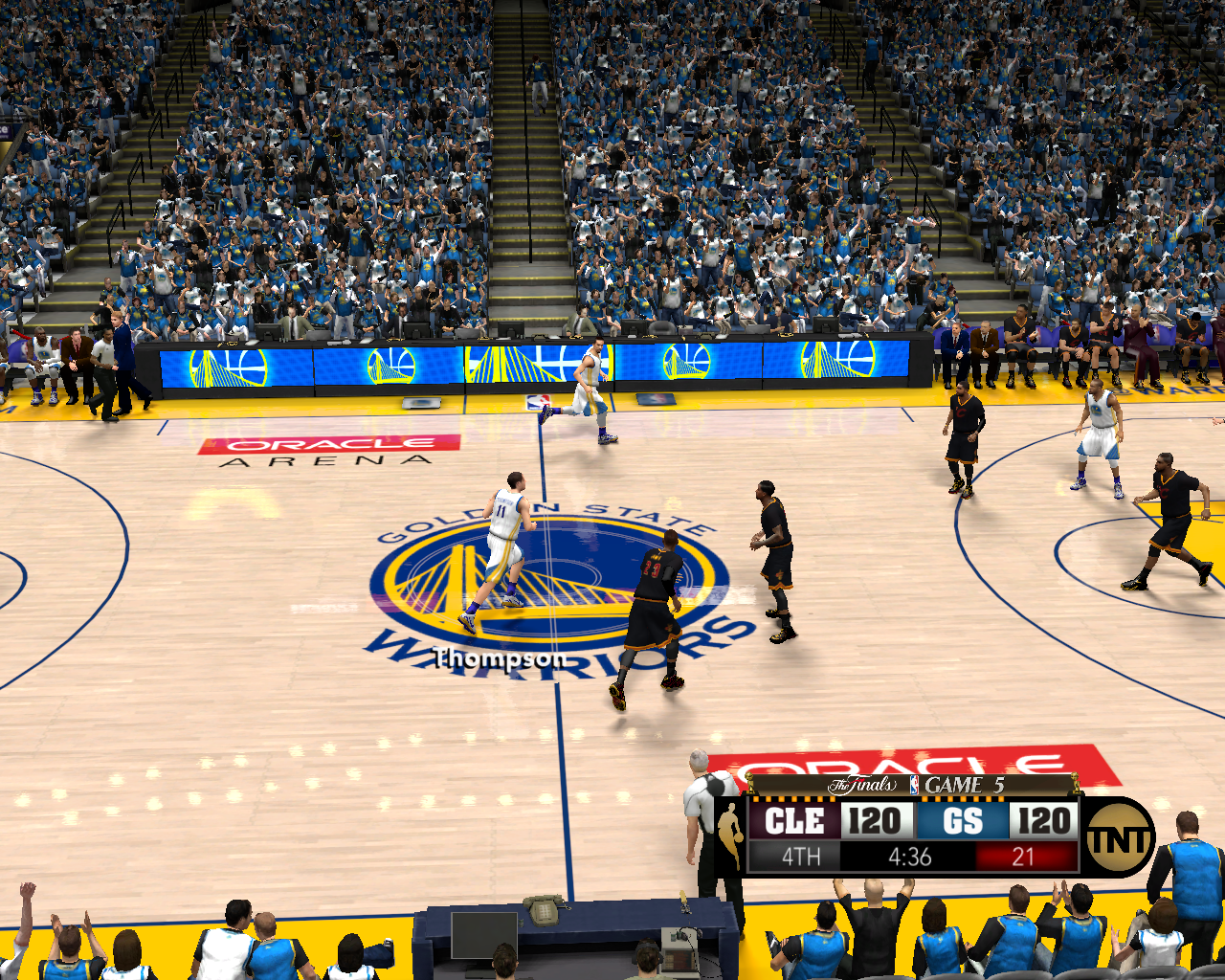This is a detailed color photograph, oriented in landscape. Taken from a vantage point high in the grandstands at mid-court, the image provides a sweeping view of a basketball court below. On the court are two teams, one dressed in dark green uniforms with gold accents and the other in white uniforms, engaged in what appears to be the final moments of an intense game. A closer inspection reveals that the players are digital, suggesting that this is a still from a video game.

In the lower right-hand corner of the image, the scoreboard displays the score: CLE 120, GS 120. The game is in the fourth quarter with the clock showing 4:35 and a smaller indicator reading 21. The top of the image prominently declares this as "The Finals, Game Five," emphasizing the high stakes of this virtual match.

The court itself is surfaced with light-colored wooden planks, accented by blue lines that outline the various sections of play. Beyond the court, the stands are filled with a digital crowd, primarily dressed in blue and white, adding to the atmosphere of excitement and anticipation.